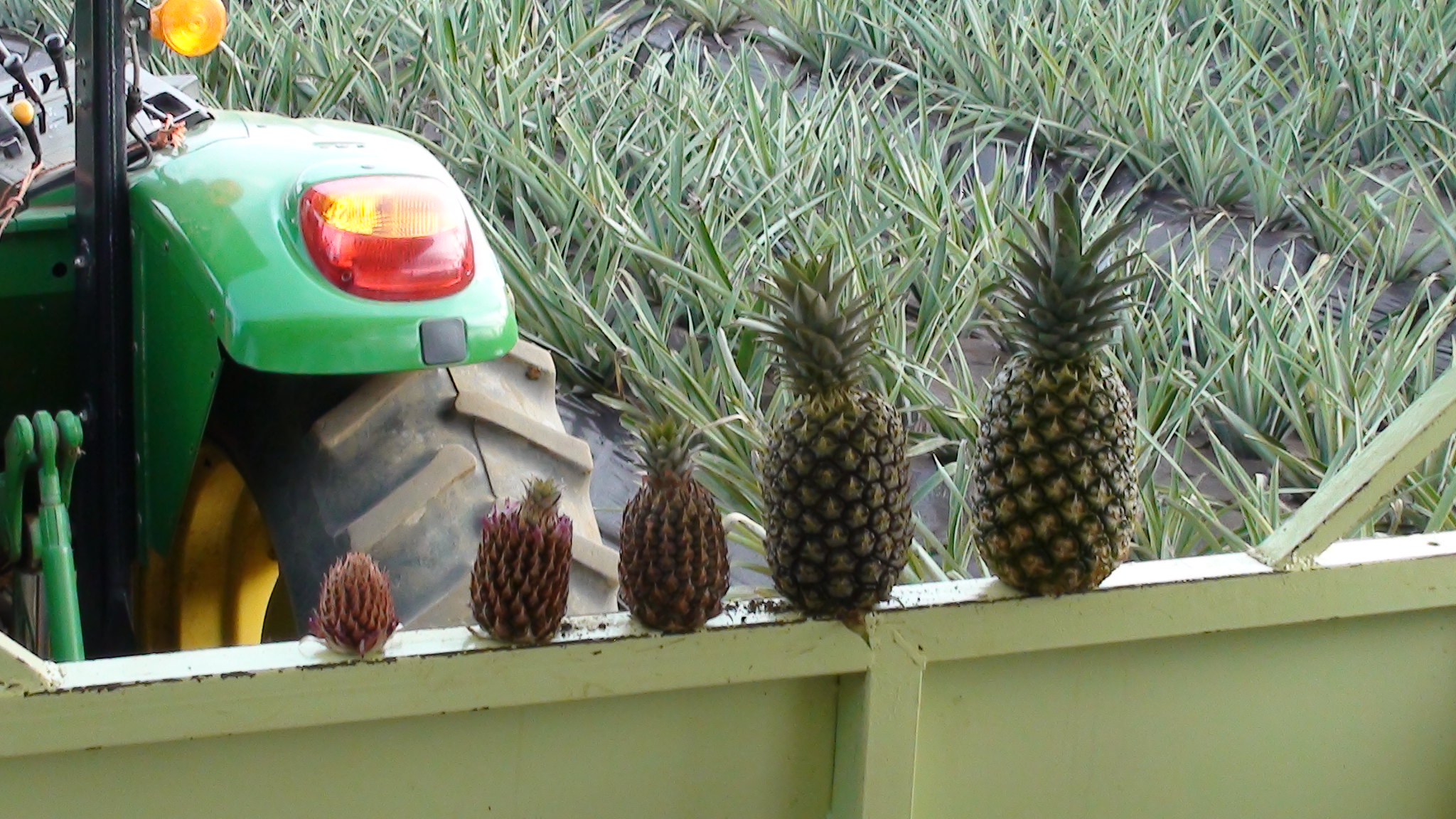This color photograph is horizontally cropped to showcase a metal wall painted in a very pale shade of yellow. On top of this wall, centered in the middle of the image, are five pineapples arranged in ascending order from left to right, starting with the smallest on the left and culminating with the largest on the right. The pineapples exhibit a light green and yellow-brown coloration. To the left side of the image, partially in the background, is a green tractor with red headlights and large rubber tires that have yellow rims. Behind the wall and tractor, rows of lush green plants or crops can be seen, possibly fixed to the soil with black plastic. The soft yellow and light green hues of the surrounding brush add depth to the background, reinforcing the impression of a bustling agricultural scene, potentially a pineapple farm.